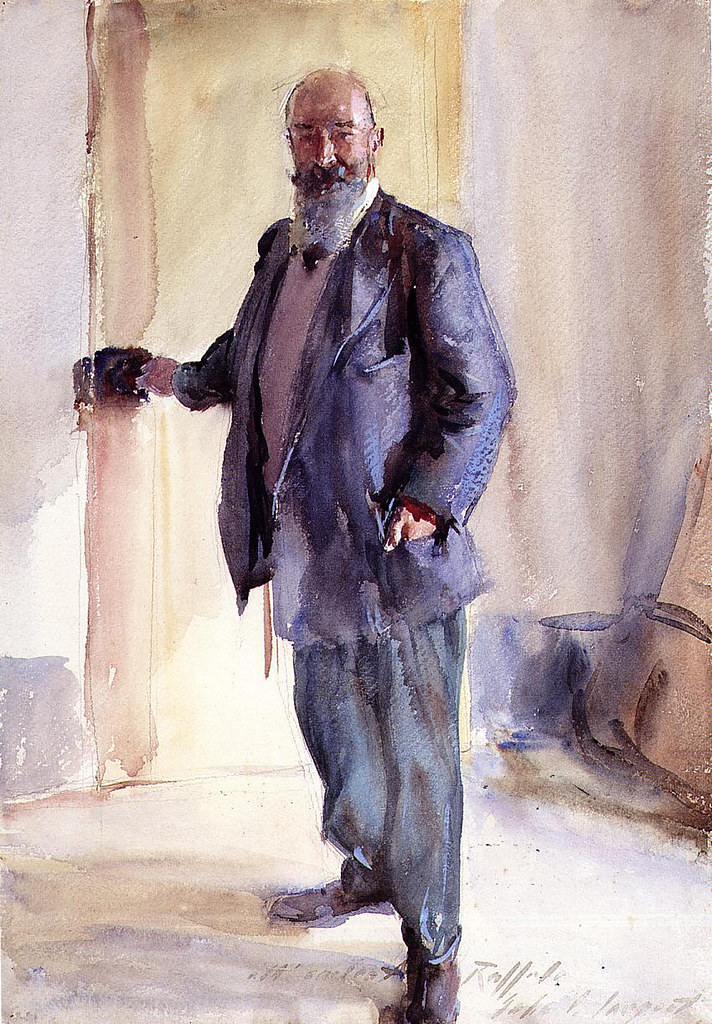This detailed painting captures an older, bald man with a long gray beard and a black mustache, dressed in a slightly oversized gray suit layered over a white sweater and collared shirt with a tie. His black shoes peek out from beneath his trousers. The man gazes at the viewer with a smile, one hand grasping a black doorknob on a yellow door behind him, as if caught in the act of opening it. The setting is a room with white, slightly discolored walls, giving it a quaint, timeless feel. The painting, which is done in oil and bears a signature at the bottom, seamlessly blends the realistic depiction of the man with subtle artistic touches.